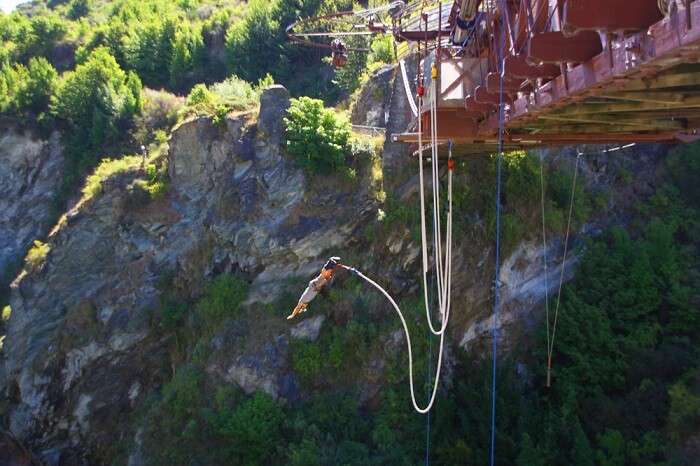In this vibrant and dynamic outdoor image, a daring individual is captured mid-bungee jump from a tall red bridge that spans the upper right corner of the scene. The jumper, who wears shorts and has their legs pointed forward while their arms are extended outward, is connected to a taut white cord looping around their ankles, suggesting they have recently leapt from the platform. The background showcases a majestic, high, and rocky mountain adorned with lush green trees and bushy foliage, stretching across the center and left of the frame. The bungee jumper’s position is slightly tilted, seemingly suspended at a 45-degree angle as they descend into the canyon below. The bright, sunny day illuminates the rugged landscape, highlighting the grey cliffs and sporadic forestation. Near the top of the image, a few spectators can be vaguely seen watching the exhilarating jump, adding a sense of scale and human element to the adventurous scene.